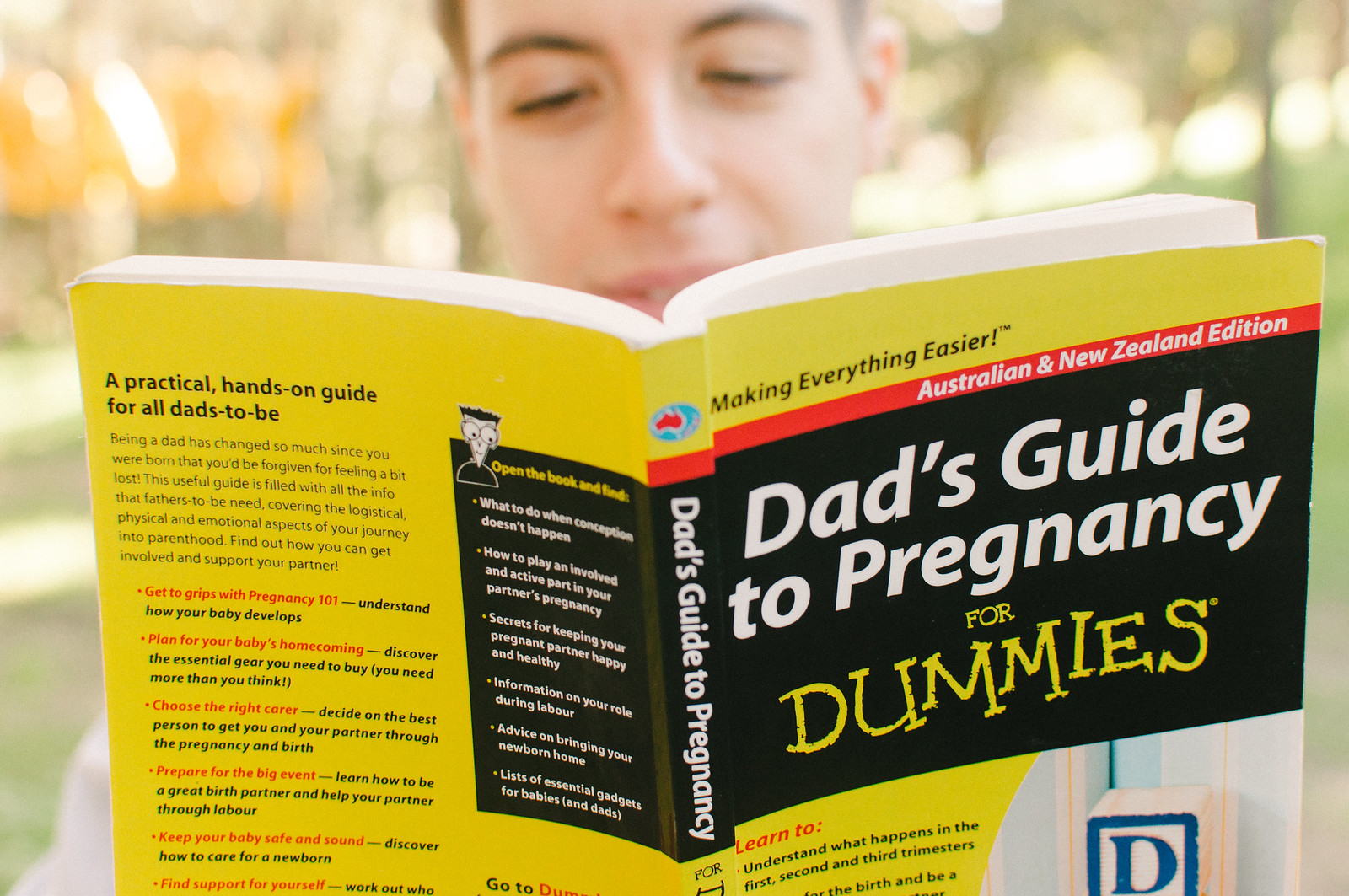A man is seen reading "Dad's Guide to Pregnancy for Dummies," and although he is out of focus, suggesting he is outdoors with blurred trees in the background, the book he holds is sharply in focus. The yellow cover of the book dominates the foreground, with a black rectangle framing the book's title: "Dad's Guide to Pregnancy for Dummies." Above this title, a red strip reads "Australian and New Zealand Edition," with the phrase "Making Everything Easier" in black text situated above that against the yellow background. The logo featuring blue and red circular elements accompanies the tagline. Visible text on the book's back cover indicates it is "A Practical Hands-On Guide for All Dads-to-Be."